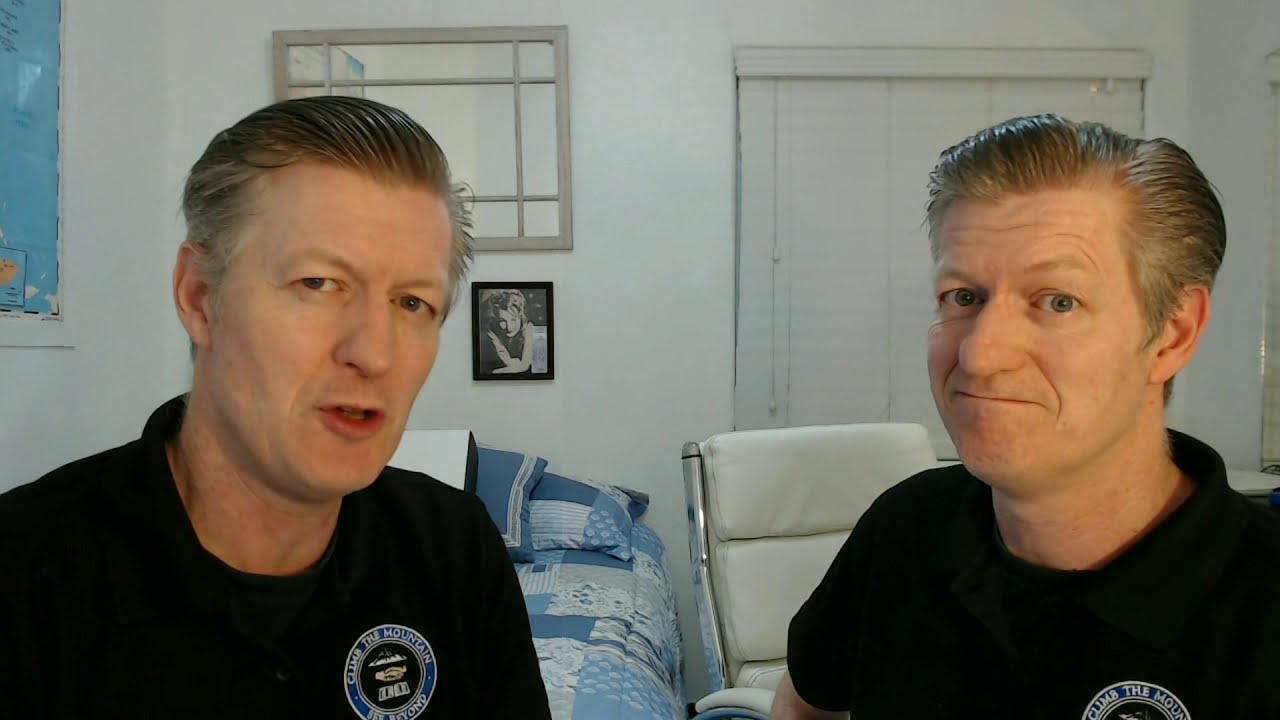In the photograph, two older Caucasian men with strikingly similar features sit side by side, suggesting they could be twins. Both have slicked-back brown hair with gray streaks and gray eyebrows. Their blue eyes gaze towards the camera, one man speaking while the other grins subtly with lips pursed inward. Each wears a black t-shirt featuring an indistinct round patch, possibly reading “climb the mountain” in white text over a blue background.

The room they are in is modestly furnished. Behind the man on the left, there is a window with blinds partially visible. A bed dressed in a blue and white quilt with pillows rests against the wall, along with a white leather chair behind the man on the right. An antique black and white framed photo of a woman hangs on the wall behind them, adding a personal touch to the otherwise simple white walls. Additionally, a map or framed piece is visible in the left corner of the image.